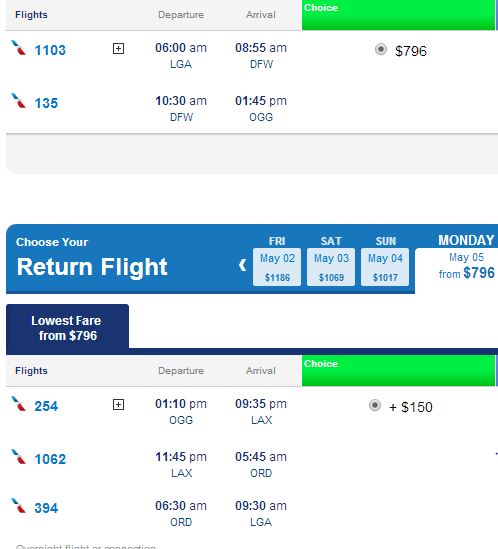Screenshot of a flight search interface showing various flight options and prices.

In the upper left corner, the interface clearly indicates the section titled "Flights." Adjacent to this, there are columns labeled "Departure" and "Arrival" in a darker gray font. A prominent horizontal green rectangle displays the word "Choice" in white.

The main section lists detailed flight information. The first entry shows a flight departing from LGA (LaGuardia Airport) at 6:00 AM, arriving at DFW (Dallas/Fort Worth International Airport) at 8:55 AM, priced at $796. The subsequent entry lists a flight departing from DFW at 10:30 AM and arriving at OGG (Kahului Airport) at 1:45 PM.

Below, a light blue horizontal heading reads "Choose your return flight," providing options for different dates and prices: 
- Friday, May 2nd for $1,186
- Saturday, May 3rd for $1,069
- Sunday, May 4th for $1,017
- Monday, May 5th starting at $796

Under these options, the section labeled "Lowest fare" offers the following flights:
- Flight 254 departing OGG at 1:10 PM, arriving at LAX (Los Angeles International Airport) at 9:35 PM for $150
- Flight 1062 departing LAX at 11:45 PM, arriving at ORD (Chicago O’Hare International Airport) at 5:45 AM the next day
- Flight 394 departing ORD at 6:30 AM, arriving at LGA at 9:30 AM

The column titles "Flights," "Departure," "Arrival," and "Choice" are reiterated here for clarity. The individual appears to be comparing flight options and prices to find the best deal.